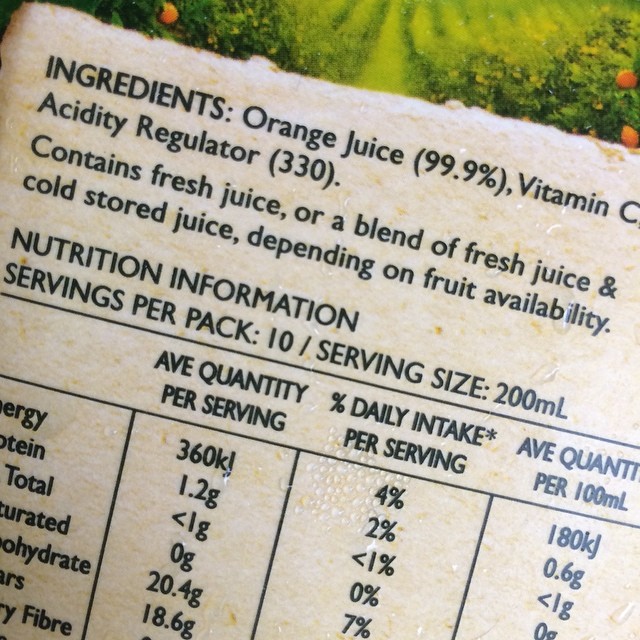The photo features a close-up of the back label of an orange juice carton, which provides detailed nutritional information and ingredients. The label prominently lists "Ingredients: Orange juice (99.9%), vitamin C, and Acidity Regulator (330)." It also specifies that the product contains either fresh juice or a blend of fresh juice and cold-stored juice, depending on availability. The nutritional facts indicate there are 10 servings per pack, with each serving size being 200 milliliters. The average quantity per serving and per 100 milliliters is detailed, including energy values of 360 kilojoules per serving (4% daily intake) and 180 kilojoules per 100 ml. Protein content is 1.2 grams per serving (2% daily intake). Total fat is less than 1 gram per serving, contributing to less than 1% of daily intake, with saturated fat being zero grams. Carbohydrates are listed at 20.4 grams per serving (7% daily intake), and sugars amount to 18.6 grams per serving. The image also shows part of the detailed rows of orange trees in a farm setting, visible at the top of the label, enhancing the product's emphasis on natural ingredients.